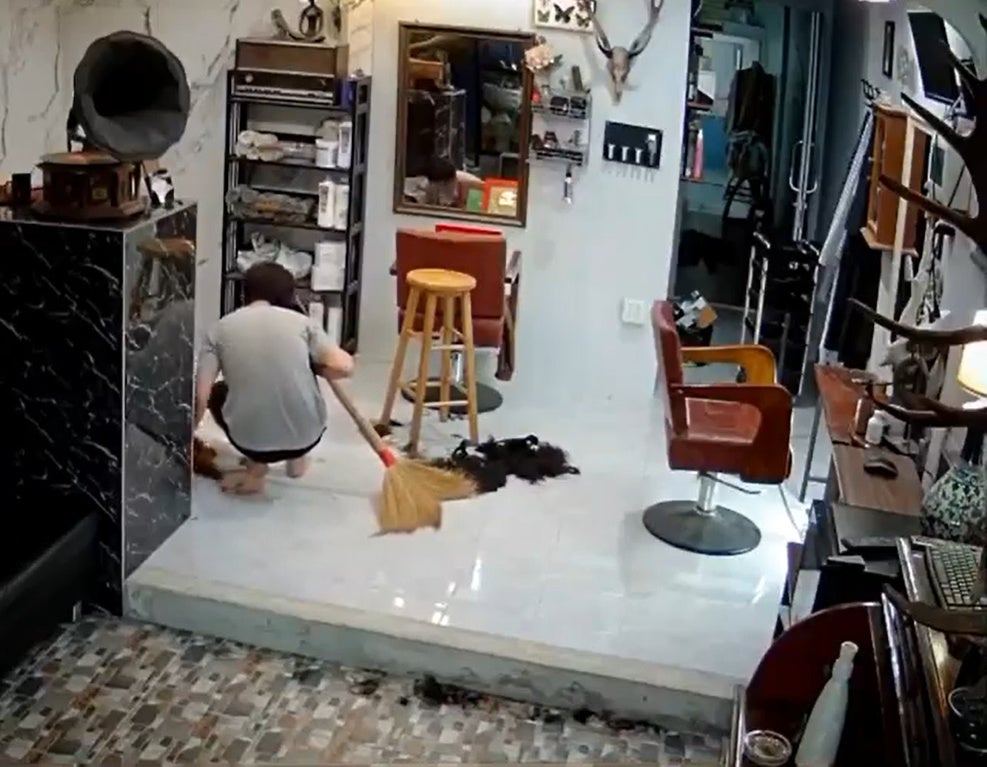The image captures the interior of what appears to be a hair salon, possibly situated in an otherwise normal house. Dominating the left side of the scene is a woman crouched down with a broom, seemingly in the process of cleaning up recently cut hair. She faces away from the camera, her task conflicting with the surrounding eclectic decor. The room features a raised marble platform and is predominantly colored in shades of white, black, and brown. 

A variety of objects clutter the space: a central stool, another barber-style chair with a metal support and brown upholstery, and a black marble pedestal with an old-fashioned radio or phonograph with a large speaker reminiscent of those seen on "Gilligan's Island." To the right, a counter or desk area holds more items, including what looks like an old typewriter, a keyboard, and a white bottle next to an ashtray. Above this desk hangs a mirror.

In the background, there's a five-shelf unit filled with various items, contributing to the room's cluttered look. Opposite the mirror sits another special hair-cutting chair. A hallway extends to the back of the room, further adding to the sense of depth and complexity in this unique and densely furnished space.